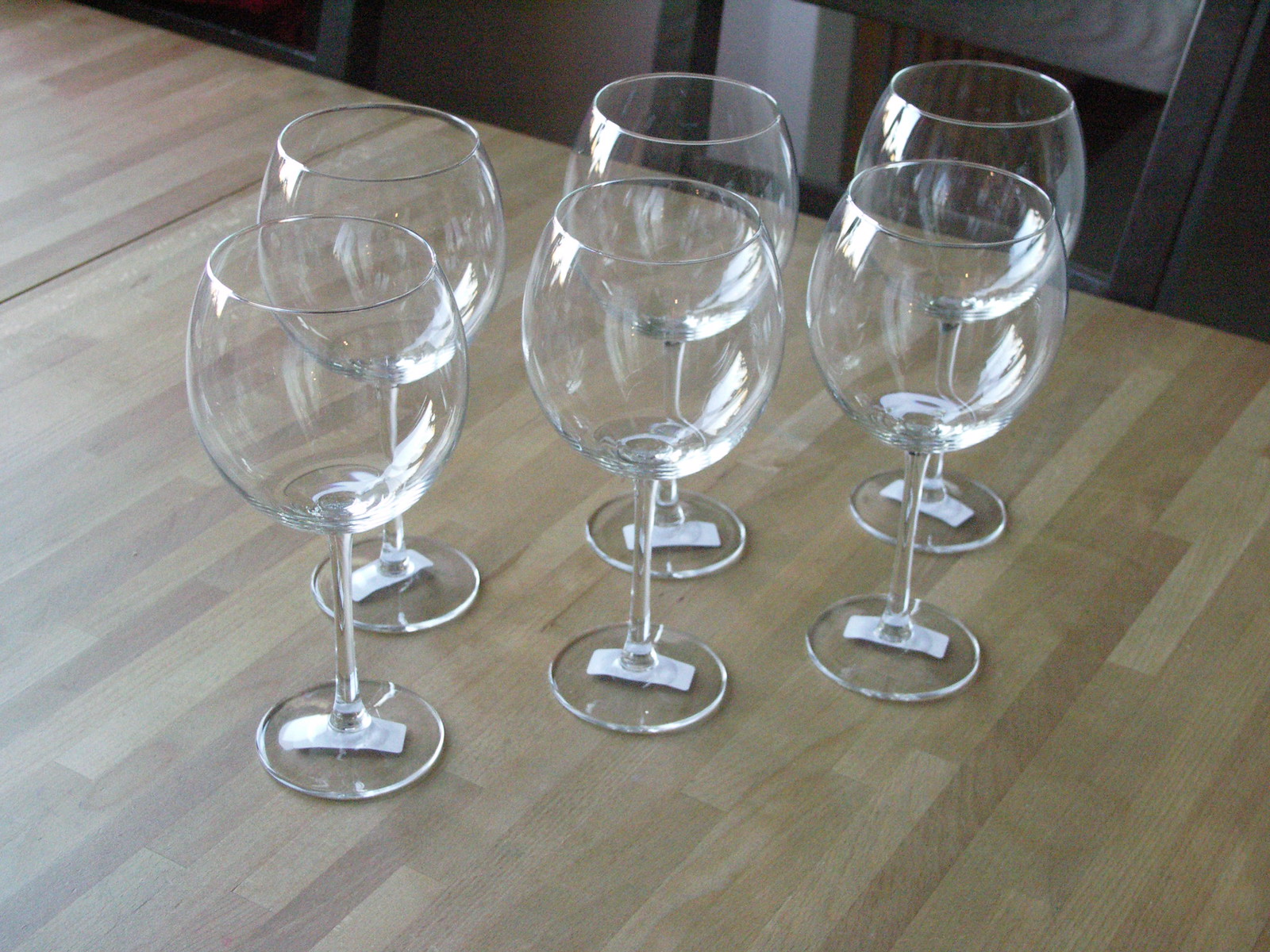The image showcases six crystal-clear, standard-shaped wine glasses arranged in a neat three by two grid at the center of a slightly wider-than-tall frame. These empty glasses feature rectangular white-backed stickers on their bases, possibly indicating price tags, suggesting they were recently purchased. They rest on a light tannish wooden table with a subtle grain pattern oriented around one o'clock. The setting appears to be indoors, resembling a dining room area, with two black, dark wooden chairs partially visible, one positioned in the upper right and another just off to the side in the upper left. Soft light from a window illuminates the bottom left corner, casting gentle reflections on the glasses, creating a serene and understated ambiance with minimal vibrancy.